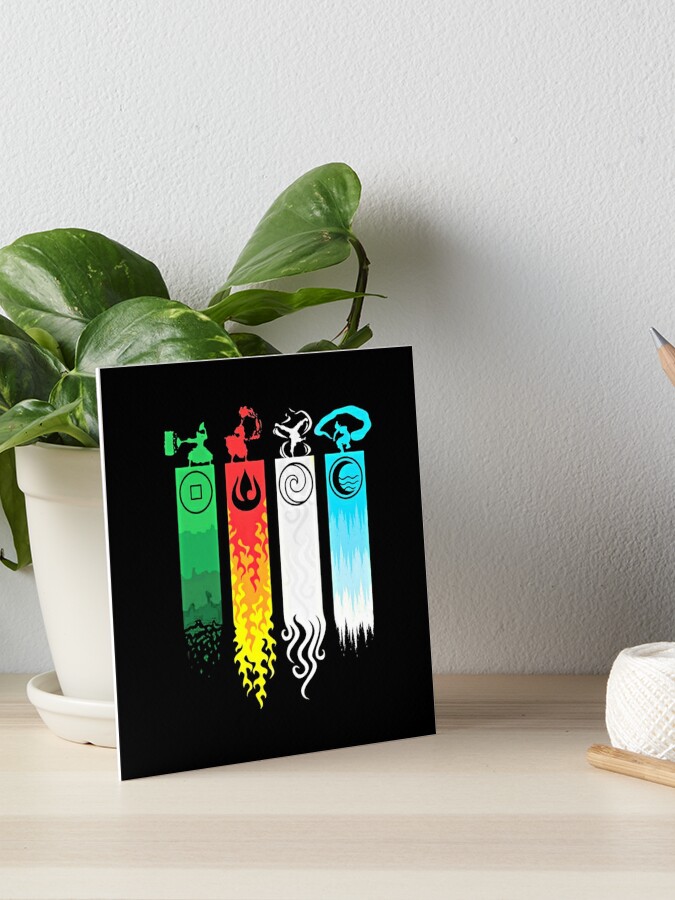The image showcases a minimalist scene featuring the stark white surface of a table with a subtle wood grain texture, set against a plain white wall. Dominating the composition is a striking black board or card, which rests against a green plant in a white pot. This black artwork features four vibrant, colored icons, each representing different figures and elements. The first icon is green and depicts a fencing person in action, while the second is a dynamic red-to-yellow gradient illustrating a fiery emblem with a fire dancer. The third icon is a pure white spiral with a gymnast performing a handstand at the top, and the fourth icon, in bright blue fading to white, appears to be a person wrapped in a long flag, evoking a circus feel. The artwork is flanked on the right side by a smaller white container holding what looks like pencils and possibly other organizing tools, adding a touch of everyday life to the artistic setup.